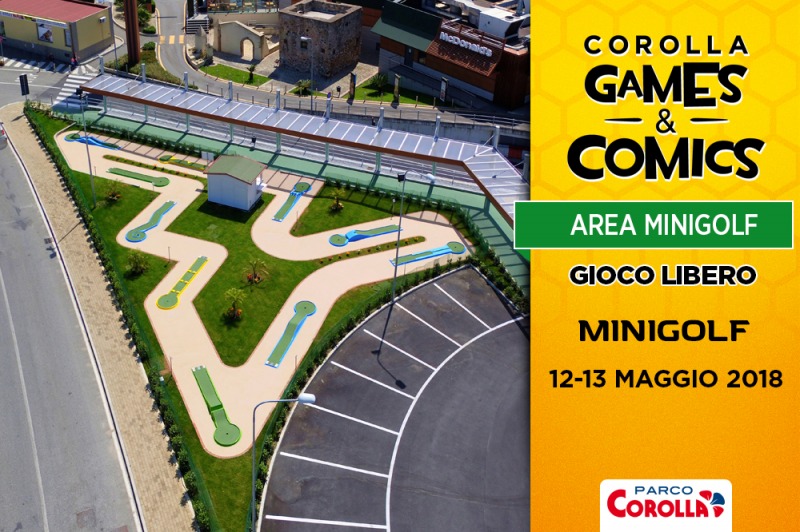The image is a rectangular advertisement for a mini-golf course, showcasing a well-designed combination of a photographic and graphic elements. On the left side, there is an aerial photograph taken from a drone, offering a detailed view of the mini-golf course. The course is surrounded by roads, including a nearby highway, and is bordered by multiple buildings, including a recognizable McDonald's.

The lush green grass of the mini-golf area is divided into various sections, with a cream-colored path weaving through the course. The mini-golf course features several holes and a small shed at the top center. The surrounding area includes a parking lot with clearly marked white dividing lines.

On the right side of the image, a vertically oriented text box with an orange-gold gradient background provides relevant information. At the top of the text box, "Corolla Games and Comics" is prominently displayed in large black text. Below it, a horizontal green strip features the words "area mini-golf" in white text. Further down, "Giaco Libero mini-golf" is listed, accompanied by the dates "12-13 Maggio 2018," suggesting a particular event or contest held during that time. At the bottom of the text box, the logo of Parco Corolla is displayed, with "Parco" in dark black text overlaid on a red design, and "Corolla" beneath it in red text. 

This advertisement effectively blends photographic realism with graphic design to provide a comprehensive and enticing overview of the mini-golf course and its amenities.